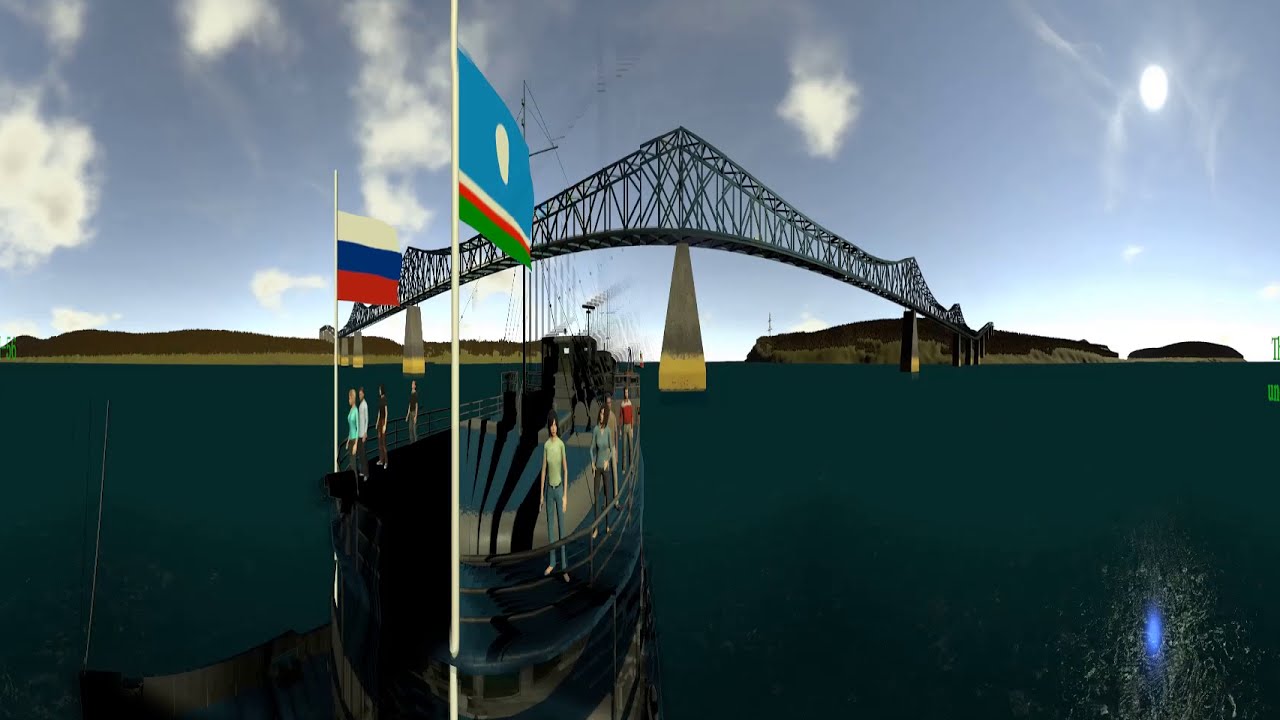In this digitally-rendered, highly detailed image, we see an elongated, distorted bridge with a prominent arch at its center, spanning between two hilly landscapes. The bridge, which appears to be made of metal and supported by pillars, stretches across what looks like a large waterway. The water beneath is depicted with a uniform shade of blue, adding to the artificial feel of the image. In the foreground, a boat approaches the viewer, manned by eight 3D-modeled figures—four on each side—against a clear yet partly cloudy sky. The boat is adorned with flags, including the Russian flag and another from an Asian-European country. The sun illuminates the scene from the right, casting a glow over the clouds and enhancing the surreal, pixelated quality of the overall picture, suggesting that this might be a scene from a video game or a computer-generated environment. The rocky outcrops on both sides of the water add to the image's authenticity, despite its digital origin.